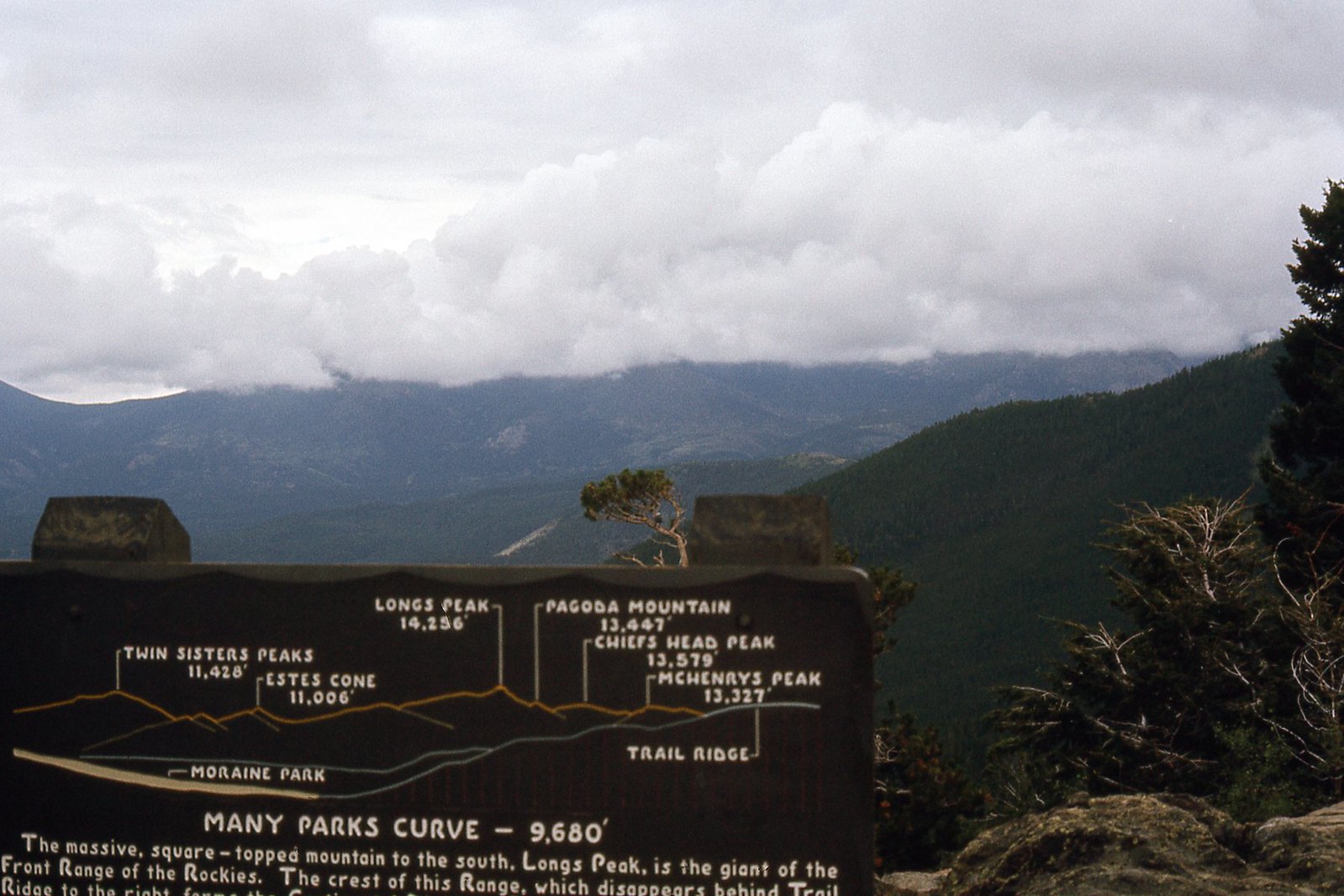This photograph, taken high in the mountains at a peak turnout, captures a breathtaking overlook of the surrounding mountain range. The scene is dominated by a mix of gray and white clouds that hang low, seemingly at the same level as the mountaintops, creating a dramatic sky. Below the clouds, the peaks of the mountains stretch out, with green slopes and dark brown tops visible, though some are partially obscured by the cloud cover. 

In the foreground, on the lower left corner, stands a partially visible, possibly wooden or metal, rectangular sign providing detailed information about the various mountain peaks visible from this vantage point. The sign lists landmarks such as:

- **Twin Sisters Peaks** at **11,428 feet**
- **Estes Cone** at **11,006 feet**
- **Longs Peak** at **14,256 feet**
- **Pagoda Mountain** at **13,447 feet**
- **Chiefs Head Peak** at **13,579 feet**
- **McHenry’s Peak** at **13,327 feet**
- **Many Parks Curve** at **9,680 feet**

There is also a trail ridge marked with a line pointing to a curved trajectory across the peaks. The lower right corner of the image features a tall pine tree along with some smaller trees and a rock, adding to the natural beauty and the serene feel of this mountain overlook. The absence of people in the shot enhances the sense of tranquility and isolation.